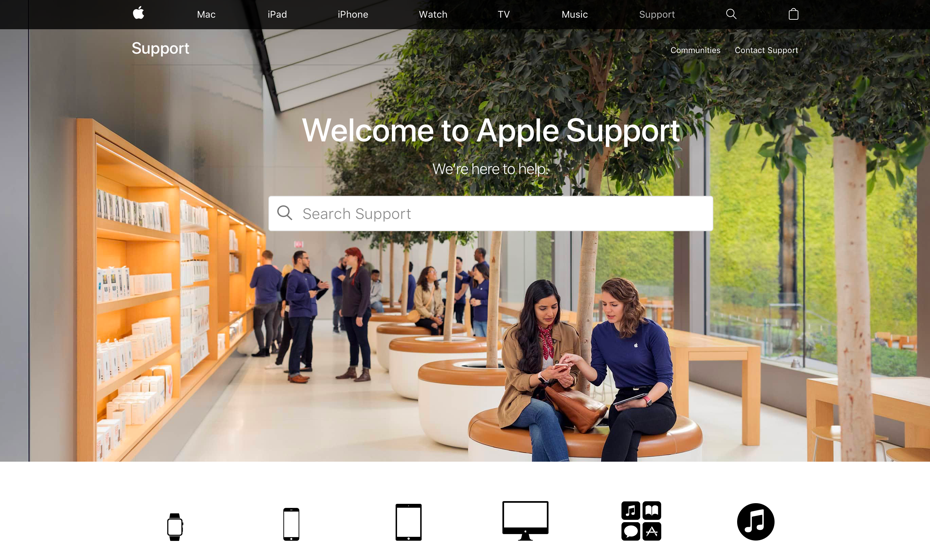This post showcases a detailed screenshot of the Apple Support website, a resource provided by the renowned tech company Apple Inc., which specializes in devices such as phones, computers, tablets, and watches. The top of the screenshot features a sleek navigation menu with clear icons and labels for various Apple products: Mac, iPad, iPhone, Watch, TV, Music, and, naturally, Support.

The main focus of the image is the Apple Support section, displaying a photo of Apple Store staff assisting customers, highlighting the company’s modern, clean, and futuristic ambiance. The store’s staff is engaged in resolving software issues, hardware damage, or other queries customers may have about their devices.

Centered in the image, there's a prominent search bar where users can type in specific issues or topics they need help with. Whether it's a software glitch or a cracked screen, this section is designed to guide users to the appropriate support resources.

Overall, the image encapsulates Apple’s commitment to providing comprehensive, user-friendly support for their entire range of products.